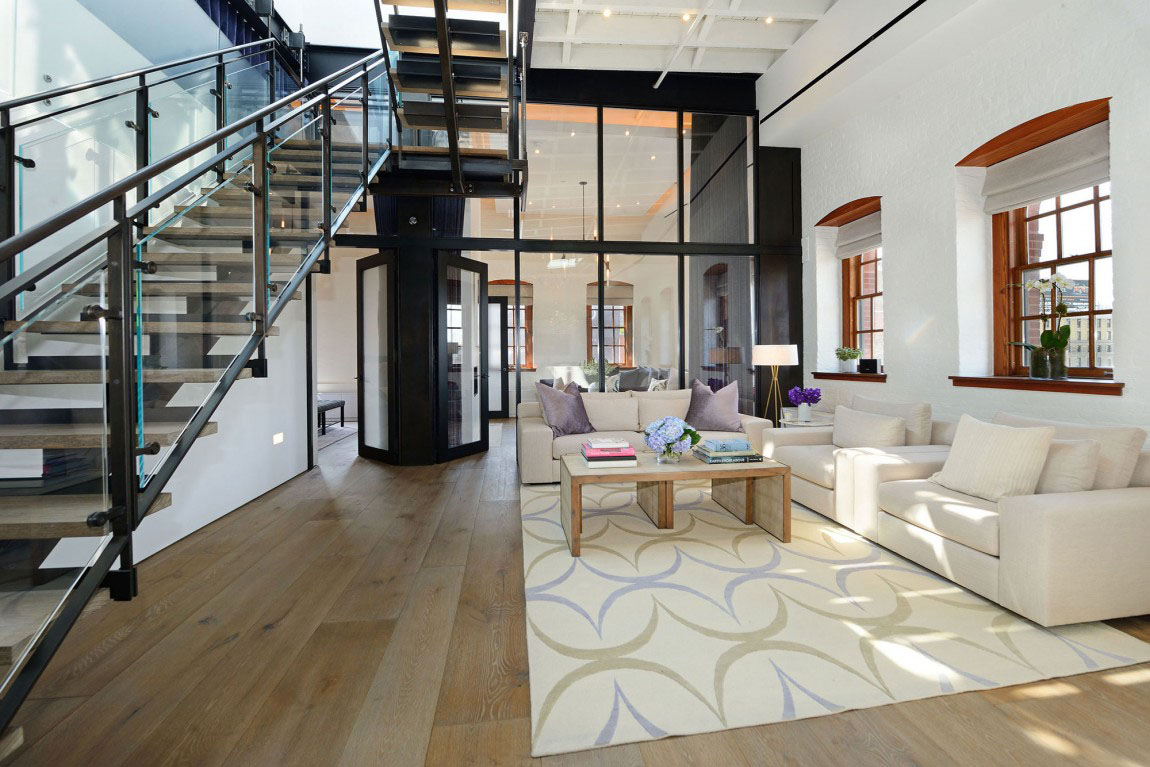The image showcases the interior of a modern, spacious living room with high ceilings, indicative of a double or one-and-a-half level room. The floor is hardwood with a white, black, and beige rug beneath three white sofas arranged around a wooden center table. The sofas comprise two couches and a love seat, forming a cozy seating area. A smaller table with books and a vase of flowers accentuates the central space. The left side features a stylish staircase with wooden steps and glass railings, split into two flights. On the right, large windows with brown frames flood the room with natural light, enhancing the bright and open atmosphere. These windows host plants in transparent and other vases. The far wall, entirely glass, offers a glimpse into an adjoining room, further showcasing the home's open-concept design.